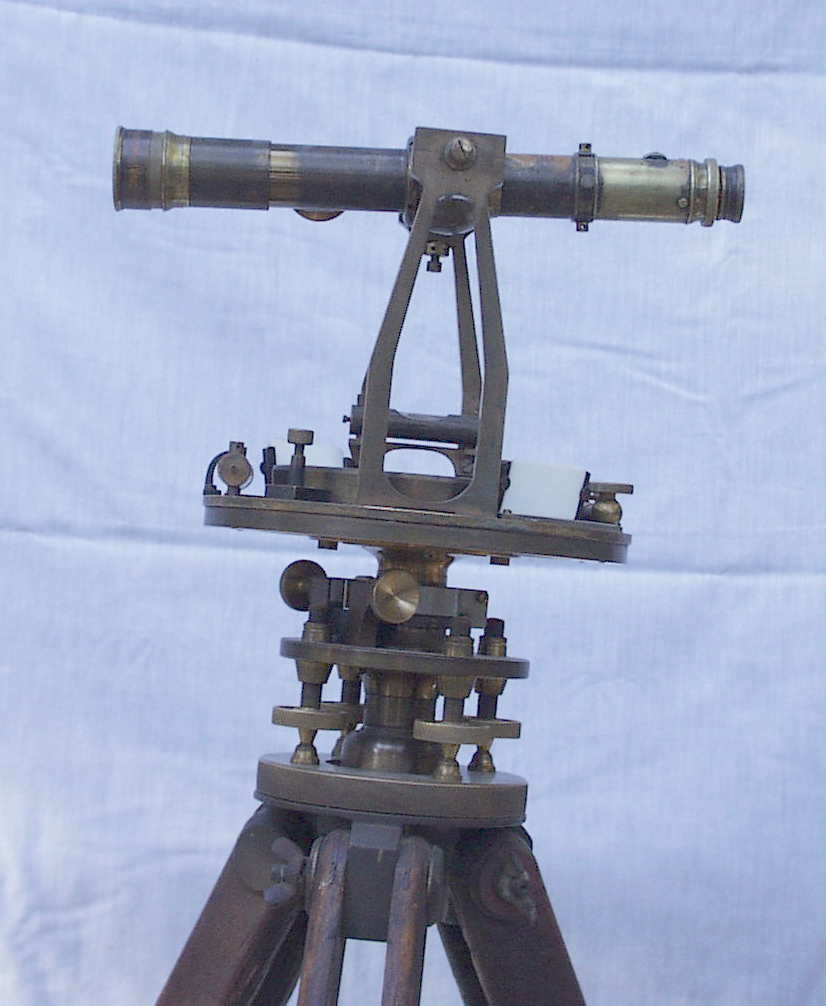The image prominently features an antique telescope positioned centrally, measuring approximately one foot in length. The telescope, made of a rustic brown or tarnished brass metal with dark bronze and black tones, appears quite worn yet well-maintained for its age. It is mounted on a tripod that shares the same color scheme and vintage appearance, though noticeably weathered. The telescope includes various brass levers and buttons, one of which seems to have been replaced due to its relatively better condition. The background is a light blue, wrinkled fabric that might appear white or stone-like, depending on the lighting and angle. The scene is devoid of any people, animals, or structures, focusing solely on the historic telescope facing left against the subdued, cloth backdrop.